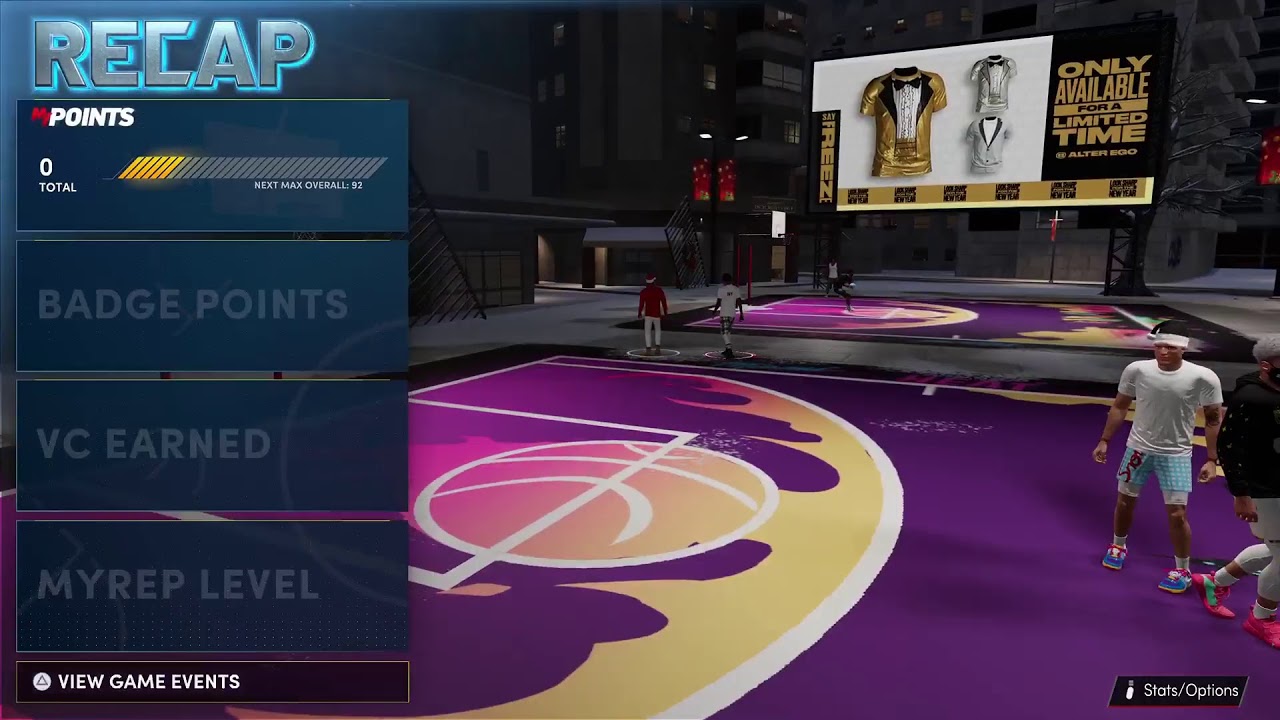This image appears to be a screenshot from a video game, likely a sports simulation. In the upper left corner, the word "RECAP" is displayed in grey capital letters with a blue border. Directly below this, there are panels indicating various totals, which are currently at zero. A progress bar, composed of diagonal lines, is predominantly yellow on the left side with the remaining section in grey. Beneath the progress bar, there is a blue rectangle with sections for "Badge Points," "VC Earned," and "MyREP Level," all of which are greyed out. 

At the bottom of the screen, white text reads "View Game Events." 

On the right side of the image is what appears to be a depiction of a stadium or sports pitch with a purple floor. Centrally located on this field is a large yellow circle bordered by a smaller yellow circle, both outlined in white, flanked by purple sections on either side. 

A player is visible to the right wearing a bandana, a grey t-shirt, blue shorts, and blue shoes. Another player can be partially seen, sporting what looks like a black top, white trousers, and pinkish shoes. Additionally, a third player is visible in the distance. 

In the background, a screen mounted on the wall displays an image of a golden jersey next to a silver item, accompanied by text stating "Only available for a limited time."